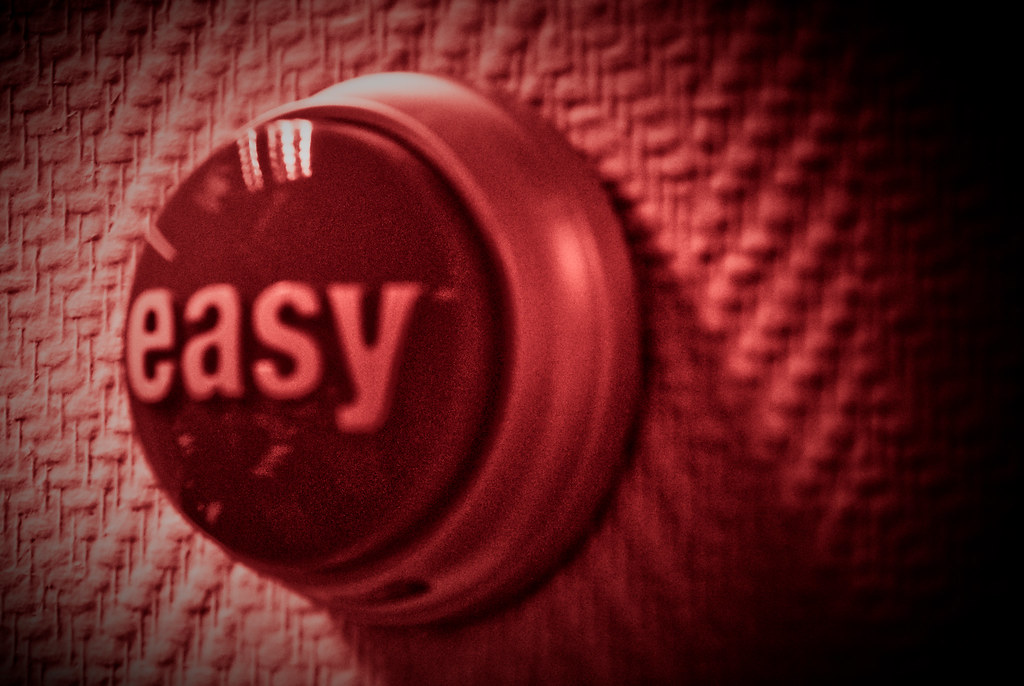The image is of a prominent button with the word "easy" in large, extruding white text. The button itself has a metallic housing, possibly with a silver outer shell, and a big black center. The entire scene is bathed in a red light, giving the image a dramatic tint. The button appears slightly dirty with small specks or tick marks illuminated, adding to its textured look. It's affixed to a panel that seems to have a rippled, dented surface, resembling woven fabric or synthetic cubicle material. The right side of the photo is notably dark, and the image appears to be lit from the left, creating a pinkish hue on that side, with black gradients in the top and bottom corners.